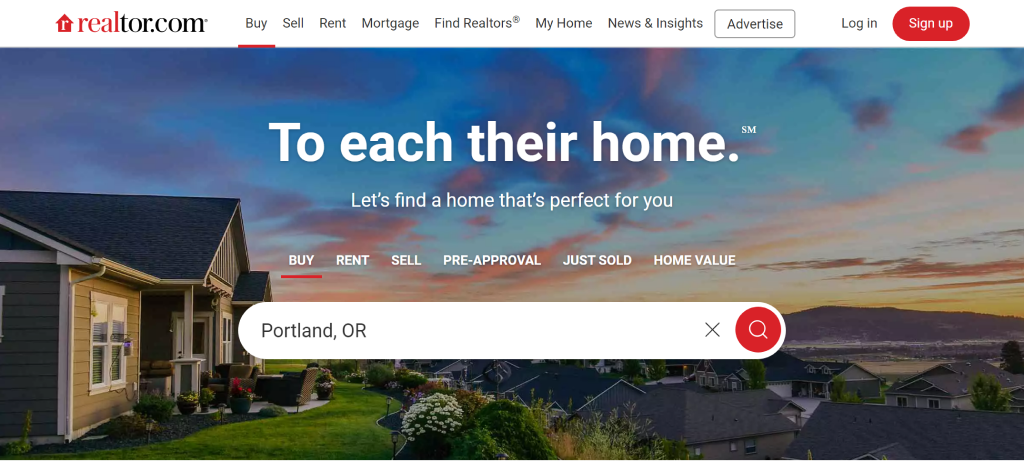The banner image on the website presents a picturesque outdoor setting. It captures a twilight sky that transitions from a dark blue on the left to a lighter blue on the right. Wisps of clouds drift through the sky, subtly tinged with pink hues. Below, a quaint house sits serenely on a hill, surrounded by a lush lawn dotted with vibrant flowers. The scene extends to a charming village nestled below, with several unique houses. In the background, a stunning sunset illuminates a rugged mountain range. The landscape is dotted with various trees and flowers, enhancing the idyllic atmosphere.

Centrally positioned in white print, the text reads: "To each their home. Let's find a home that's perfect for you. Buy, rent, sell, pre-approval, just sold, home value." 

Below this, a search engine field is prominently displayed, pre-filled with "Portland, Oregon." Adjacent to the field, a red circle encloses a white magnifying glass icon. At the top of the banner, the Realtor.com logo is prominently placed, followed by navigation options: buy, sell, rent, mortgage, find Realtors, my home, News & Insight, advertise. The options to log in and sign up are highlighted in red with white text.